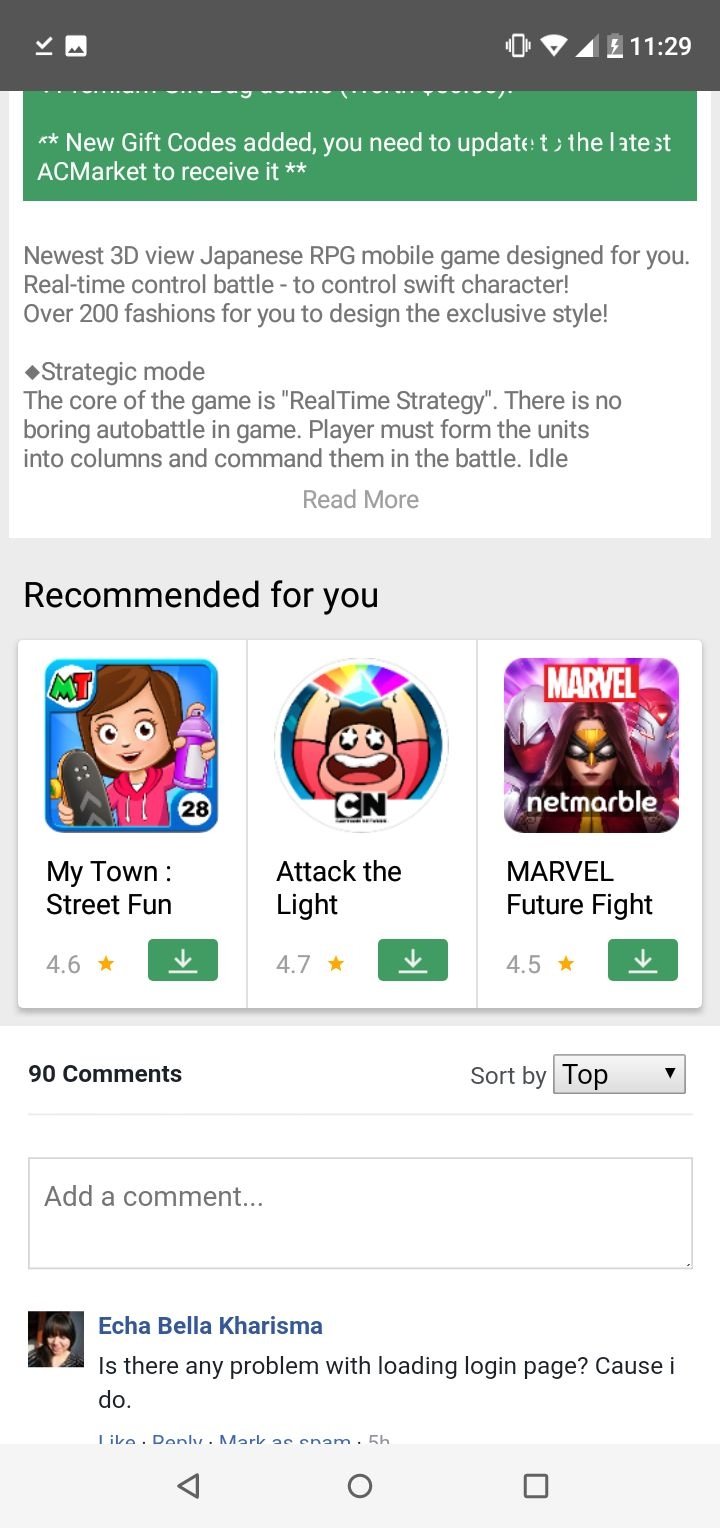**Caption:**

The image appears to be a screenshot of a smartphone screen. At the top, a dark gray bar shows typical phone icons. The time displayed is 11:29. Below this, there's a prominent green box with white text, featuring a star symbol, which reads, "**New Gift Codes Added**. You need to update to the latest AC Market to receive it," flanked by two additional stars.

The main content area is against a white background, featuring gray text that announces: "Newest 3D view Japanese RPG mobile game designed for you. Real-time control battle to control swift characters. Over 200 fashions for you to design the exclusive style." A gray diamond symbol follows this with the word "Strategic mode" next to it. The game description emphasizes, "The core of the game is 'Real-time strategy'. No boring auto battle in-game. Players must form the units into columns and command them in real-time battle." Below this, the text "Read More" is centered.

Further down, a gray box is titled "Recommended for You" in black text. Three game recommendations are shown below in separate smaller panels:

1. **"My Town Street Fun"** with a 4.6 rating, displaying an image of a little girl holding what appears to be a gray sandal and a pink spray can.
2. **"Attack the Light"** with a 4.7 rating, featuring a character in a red shirt with arms raised.
3. **"Marvel Future Fight"** with a 4.5 rating, showing a Marvel character with the text "Marvel" at the top and "Netmarble" at the bottom.

The section ends with "90 comments" and "Sort by Top," followed by a comment box. Below, a comment from user **Echa Bella Charisma** reads, "Is there any problem with loading login page because I do."

**Note:** Certain inaccuracies or ambiguities in the original description were interpreted to provide more clarity.